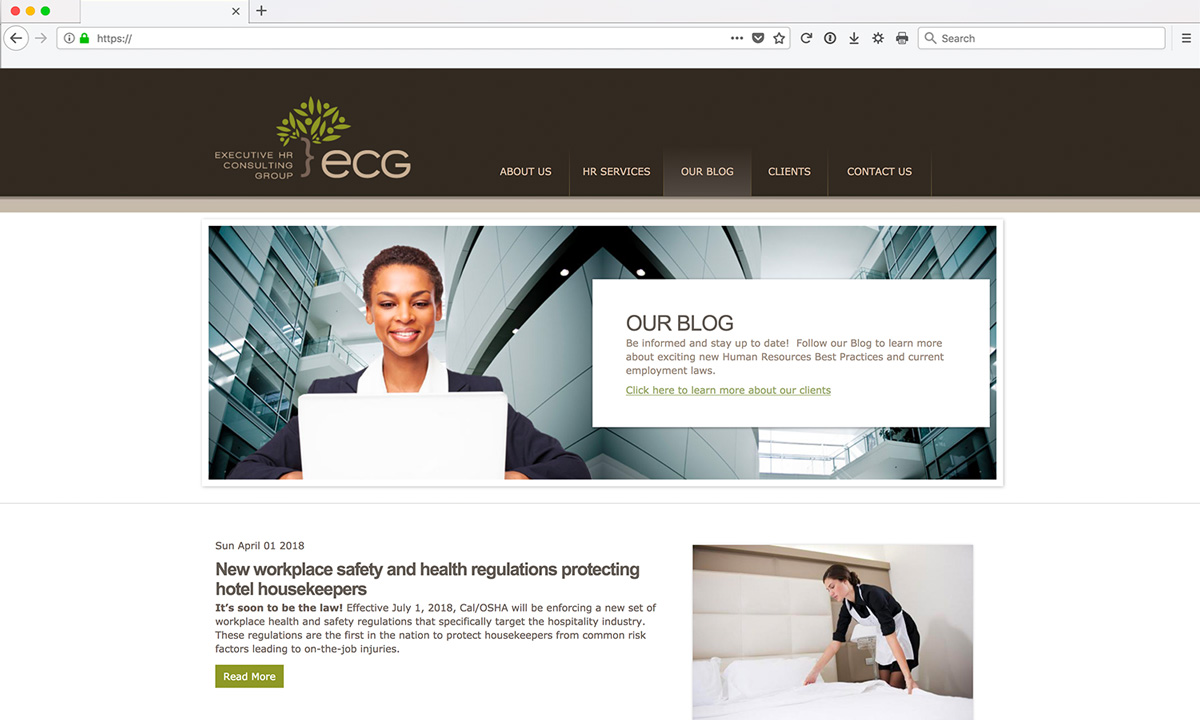The image depicts a website interface with a gray border at the top. Within this border, there are three dots colored red, yellow, and green. Adjacent to these dots are a back arrow and a forward arrow, followed by an address bar displaying "HTTPS://", but no specific URL. Moving further to the right, there are several functional icons including favorite buttons, refresh, download, a cogwheel, a print icon, and a search bar located at the far end.

Below the gray border is a section with a brown background displaying the title "Executive HR Consulting Group" alongside a small image of a tree with green leaves, accompanied by the letters "ECG" in lowercase and a tan color. The same tan color is used for the menu text on the right side of the page with options: About Us, HR Services, Our Blog, Clients, and Contact Us, with "Our Blog" highlighted.

The central content features an image of a young Black woman with short brown hair, dressed in a blue and white business suit, working on a laptop. The heading "Our Blog" is prominent, followed by the text: "Be informed and stay up to date. Follow Our Blog to learn more about exciting new human resources, best practices, and current employment laws. Click here for more information about our clients."

Below this, the text "Sunday, April 1, 2018" is displayed, introducing a blog post titled "New Workplace Safety and Health Regulations Protecting Hotel Housekeepers." The text explains that effective July 1, 2018, Cal/OSHA will enforce new workplace health and safety regulations specifically targeting the hospitality industry. These regulations are the first nationwide to protect housekeepers from common risk factors leading to on-the-job injuries. A green "Read More" button is also present.